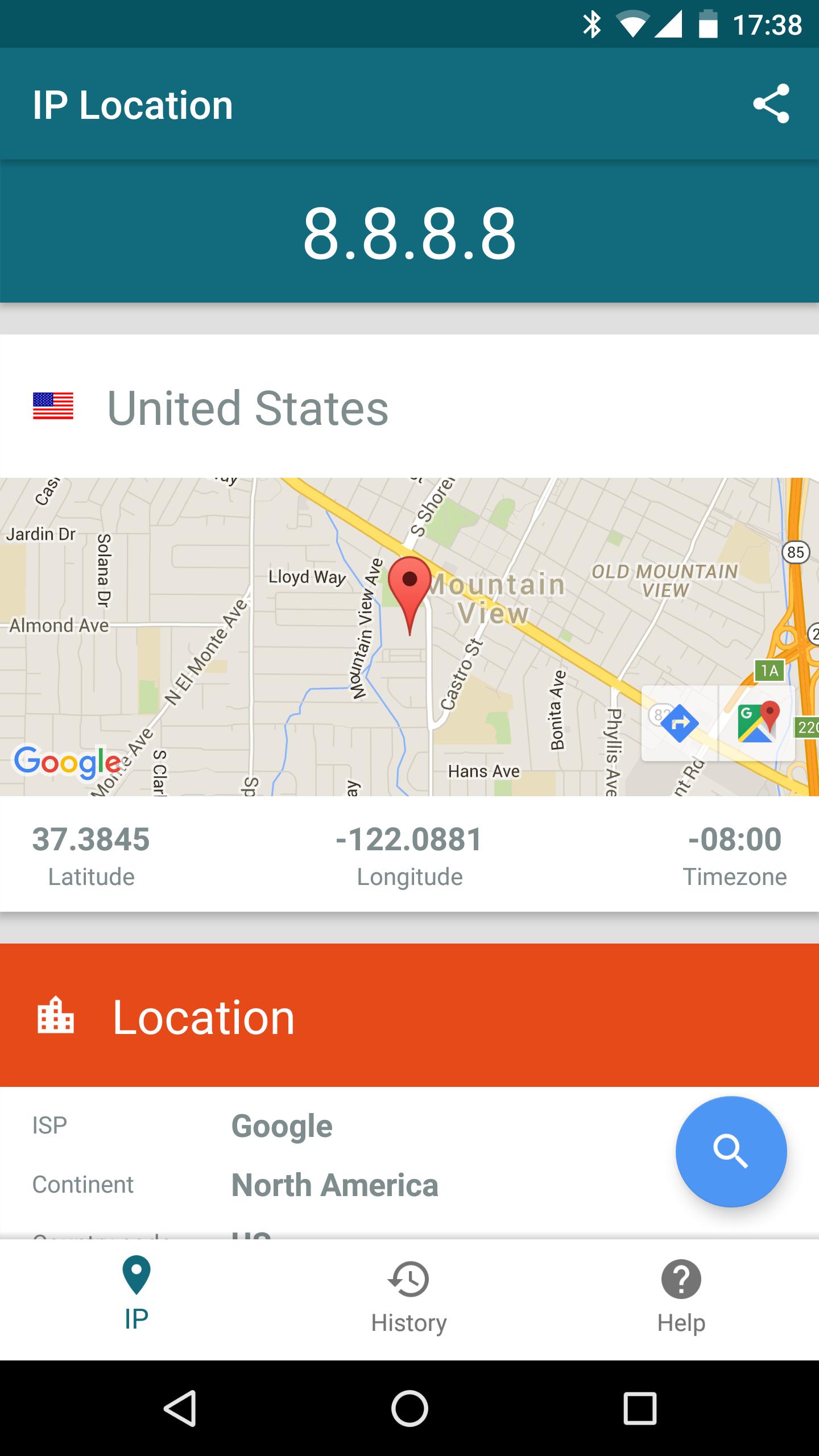This image is a screenshot from a cell phone displaying the results of an IP address lookup. The interface is visually segmented using various colors and banners for clear navigation and representation of information.

At the topmost section, there is an almost black, thin banner containing icons that indicate the phone's connectivity status including Bluetooth, Wi-Fi, signal strength, battery level, and the current time. Directly below, a dark teal banner prominently features "IP Location" on the left side. On the right side of this banner, there is an icon resembling an open crocodile mouth formed by three dots connected with lines.

The central section of the screen displays the looked-up IP address "8.8.8.8" in large, white text against a dark teal background. Below this, a white bar contains the American flag on the left and "United States" on the right, indicating the geographic location of the IP address.

Following this, a map with a pinpoint marks specific coordinates: latitude 37.3845 and longitude -122.0881, along with the time zone notation of -0800. The next segment transition is distinguished by a thin gray line.

The subsequent banner is dark orange, adorned with a factory-like symbol in white on the left, next to the text "Location." Below this, there is a white information box labeled "ISP" on the left, revealing that the IP address is associated with Google in the center of the box. Underneath, another label indicates the continent as "North America." On the far right, a blue circle with a white magnifying glass icon suggests a search feature.

Finally, the bottom section features a white bar with three icons: a pin symbol labeled "IP" on the left, a clock with a backward circle labeled "History" in the center, and a circle with a question mark labeled "Help" on the right. The very bottommost part of the screenshot shows the standard navigation bar of the phone, including a white triangle pointing left, a circle, and a square.

This detailed depiction offers a comprehensive understanding of the layout and elements present in the screenshot.